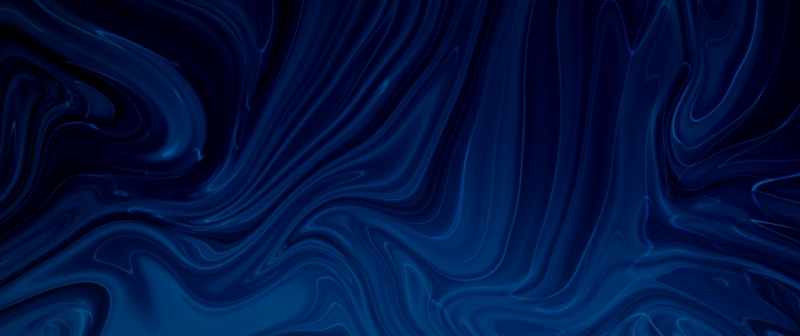The image presents a narrow, rectangular design with a rich, dark blue background and dominant, swirling wave patterns. These swirls predominately consist of softened and blurred white and varying shades of blue lines, suggesting a motion-like effect. The left side of the image starts with a very dark blue shade that transitions into hints of light blue, particularly noticeable at the bottom where it creates an impression of a wave moving across from left to right. The top portion showcases more vertical waves, which blend together with the patterns at the bottom as they move toward the right end. The overall effect of the swirls against the dark background gives a sense of depth and fluidity, reminiscent of brush strokes or smoke in the sky, evoking a calm and soothing atmosphere ideal for use as a wallpaper.